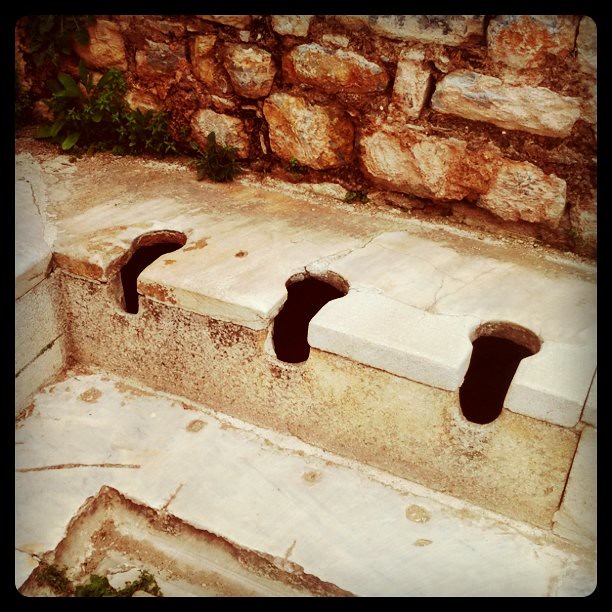The image features an ancient and abandoned structure that appears to be part of a Greek or Roman archaeological site, potentially a public bath or communal toilet area. The focal point is a stone bench-like surface with three intriguing keyhole-shaped openings. These openings have a round portion on the flat surface, which then extends as an oblong curve over the front edge onto the vertical surface below. The bench is made of solid, white marble and is situated in front of a mortared stone wall composed of various-sized rocks, interspersed with reddish mortar. The wall, along with running along both sides of the scene, adds to the historic feel. Weeds are sprouting from the base of the wall, particularly in the upper left corner of the image. The foreground showcases stepping stones and a triangular brown marking near the lower edge, with a horse-shaped marking in the middle, further accentuating the ancient and worn nature of the site. Overall, the setting conveys a sense of antiquity, abandonment, and historical significance.